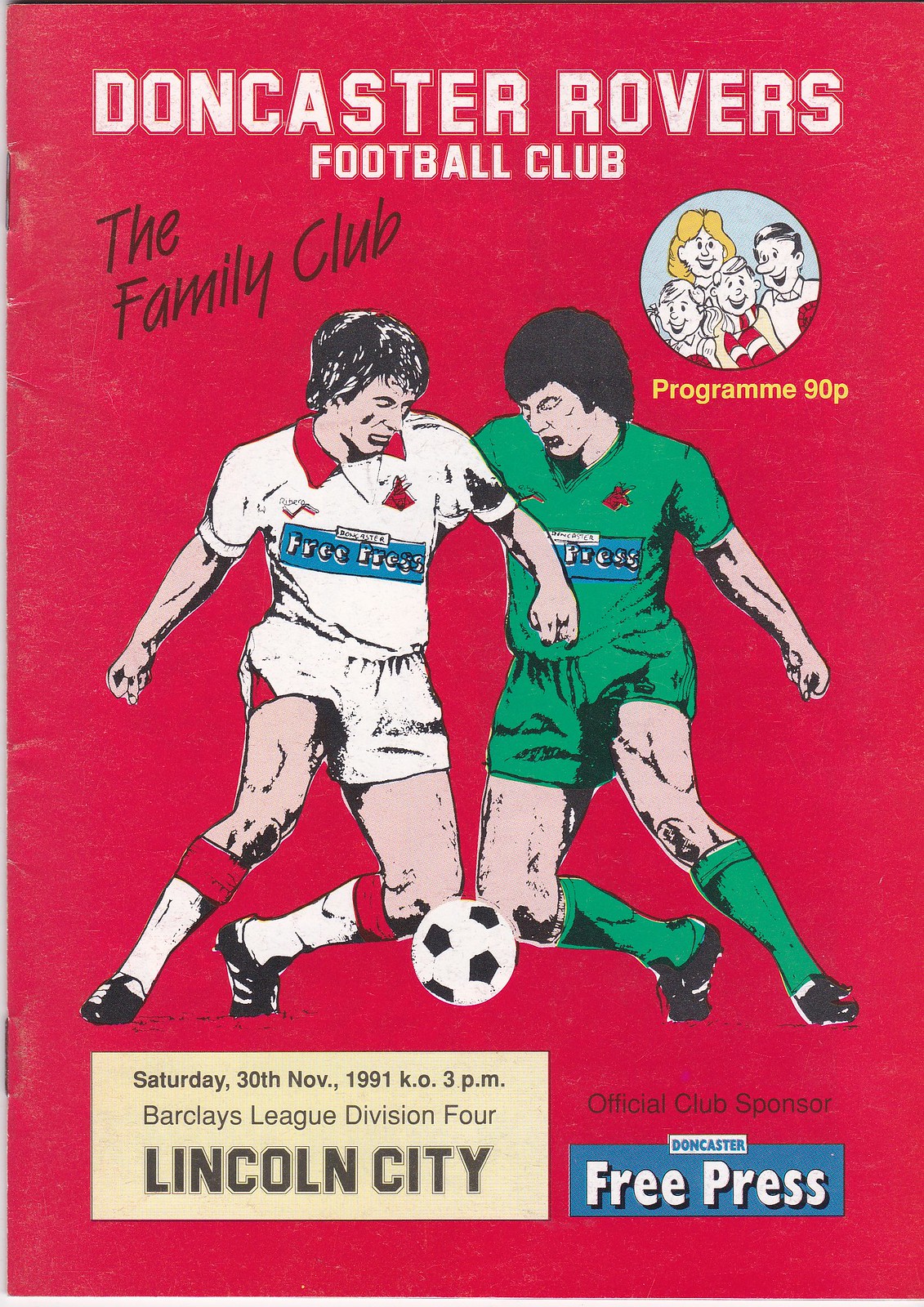The image is a vintage program cover for the Doncaster Rovers football club, dating to Saturday, 30th November 1991, with a kickoff at 3 p.m. for a Barclays League Division IV match against Lincoln City. The program is priced at 90 pence and prominently displays "The Family Club" slogan on the upper left. Dominating the center are two illustrated Caucasian football players, one in green and the other in white, engaged with a black and white soccer ball between their feet. The player in white sports red and white socks, while both have their club sponsor, Doncaster Free Press, emblazoned on their jerseys. Above the program details is an illustration of a delighted family—mom, dad, daughter, and son—emphasizing the club's family-friendly atmosphere.